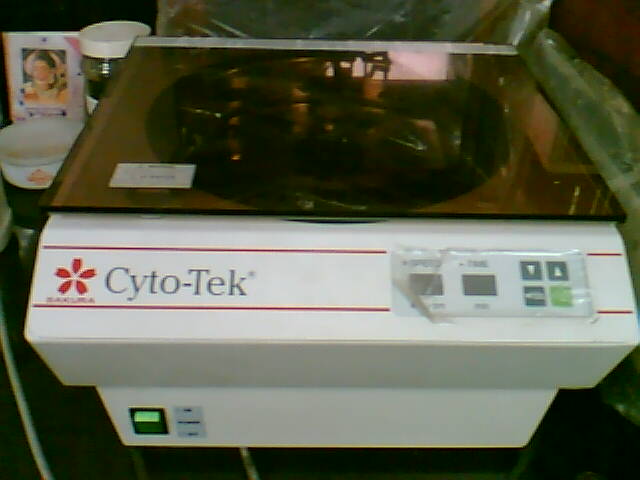The image features a worn medical device named Cytotec, which appears to be a home dialysis machine. The front of the white machine prominently displays the name "Cytotec" in gray with capitalized "C" and "T," positioned between two red lines. Beneath the logo is the maker's name, written in red. The machine has a distinctive brown, glass-like covering at the top, housing a round object. The plastic that encases some of the controls and buttons on the right side is frayed, indicating heavy use. A green on/off switch is located toward the bottom of the device. Various cords are attached to the machine, which also has a nearby jar and a small photograph contained in another vessel.